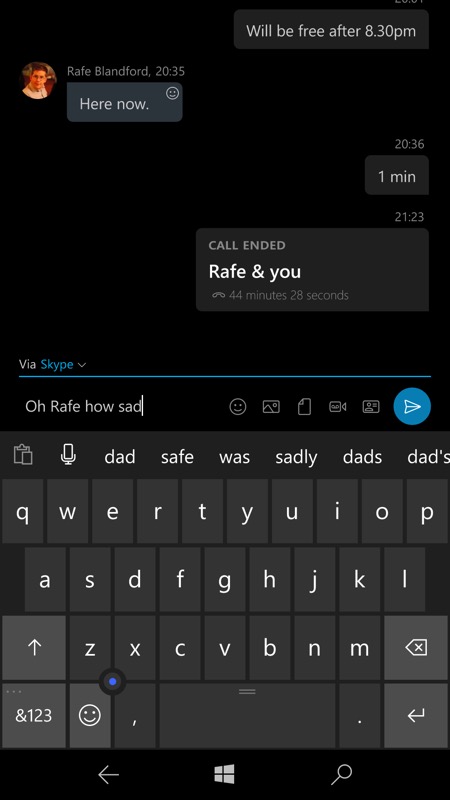### Detailed Caption:

The screenshot captures a mobile phone interface with a black background, indicating the device is in dark mode. The application in use is Skype for messaging. 

1. **Top Section**: The top part of the image shows the black background of an open Skype chat window.
2. **Messages**:
   - The initial message from the user reads, "will be free after 8:30 p.m.”
   - Rafe Blandford replies at 20:35 with the message, "here now :)".
   - At 20:36, the user responds with "one minute".
   - At 21:23, there is a notification bubble stating, "call ended, Rafe and you. 44 minutes and 28 seconds."
3. **Typing Field**:
   - Below the call notification, there's a blue line indicating the end of the chat session with “via Skype” written above it.
   - The user is currently typing in the text field, which displays the message "Oh, Rafe, how sad."
   - To the right of the text field are various icons: a smiley face emoji, a picture emoji, a piece of paper emoji, a video camera emoji, a portrait emoji, and a blue circle with a right-pointing arrow (send button).
4. **Auto Complete Suggestions**:
   - Below the text field, a gray suggestion bar offers autocomplete options for the word "sad," including "dad safe," "was sadly," and "dad's dad."
5. **Keyboard**:
   - The bottom section of the screenshot shows a QWERTY keyboard, which the user is using to type their message.

This comprehensive description captures the essence of the Skype messaging interface on a mobile phone in dark mode, detailing the conversation flow, the user interface elements, and the context of the messages exchanged.